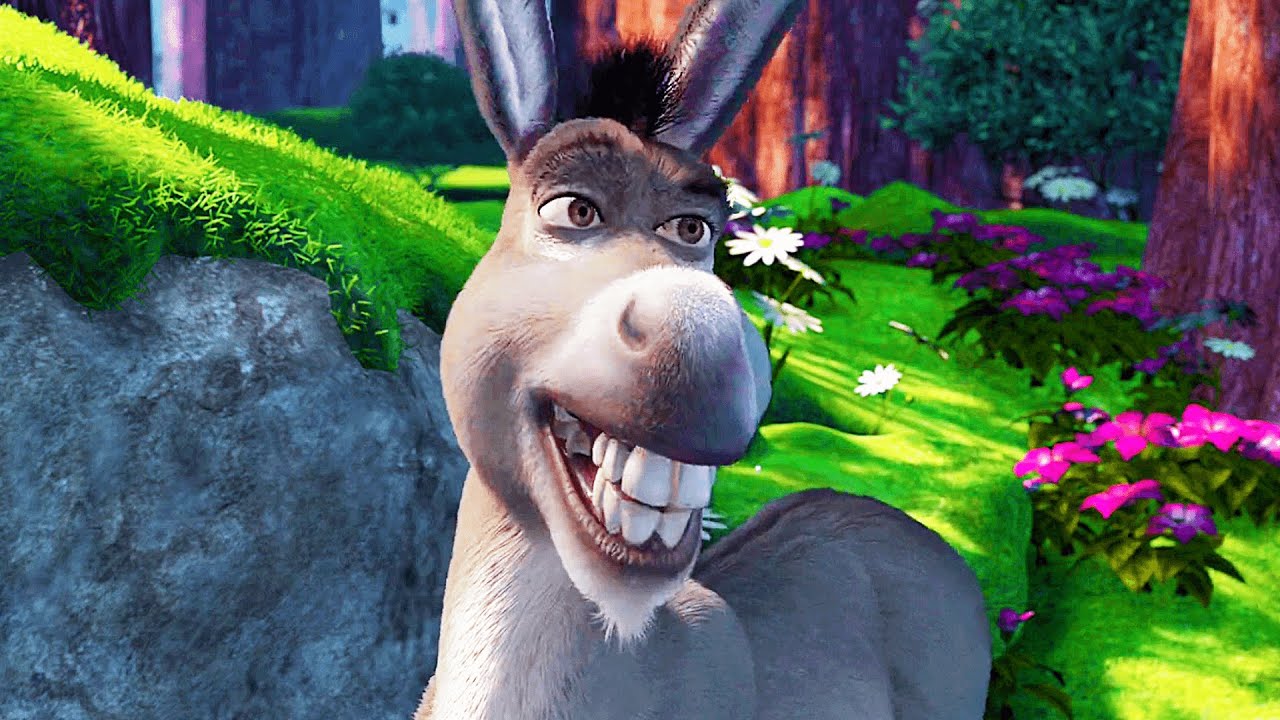This detailed image is a still shot from the animated film *Shrek*, featuring the character Donkey. Donkey is shown in vivid detail; he has a realistic appearance with a light gray fur coat, a tuft of black hair atop his head between his two large ears, which are blackish gray with white inner fur. His hazel brown eyes are wide open with dark black eyebrows above, and his lips are black with a contrasting white beard. Donkey's head is tilted slightly to his left (right from the viewer's perspective), and he is smiling broadly, showcasing his large, gleaming white teeth.

The background sets a lush, vibrant scene of a forest. Surrounding Donkey are multiple elements, including large gray rocks, some covered in moss. Bright green spring grass fills the foreground, dotted with an array of flowers—purple ones with white centers, bright white daisies with yellow centers, and fewer pink and yellowish flowers. Additionally, there are purplish-brown tree trunks, large leafy green bushes, and shrubs behind Donkey, subtly hinting at a sunlit ambiance. This composition creates a rich, enchanting environment where Donkey's playful and cheerful demeanor stands out.